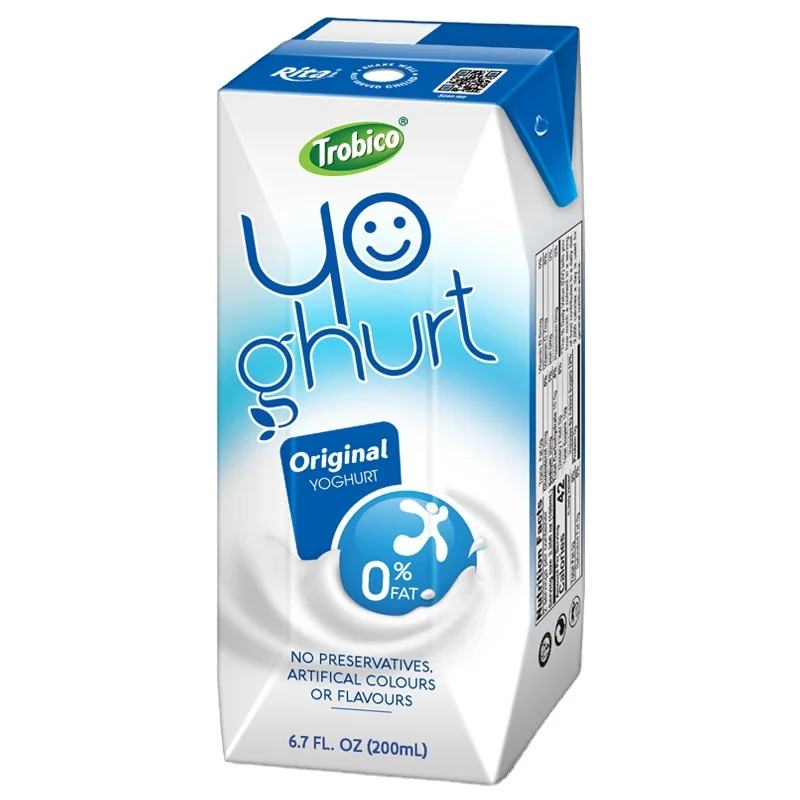The image depicts a carton of yogurt from the brand Trobico. At the top of the packaging, the brand name "Trobico" is displayed prominently within a green oval, featuring white text and accompanied by a registered trademark symbol. Below the logo, the word "yogurt" is creatively arranged on two lines— with "yo" on the first line and "gurt" on the second. Notably, the 'o' in "yogurt" is stylized as a smiley face, and the 'g' is adorned with two small leaves emerging from its top.

Directly beneath the word "yogurt," a small blue square contains the text "original yogurt." Adjacent to this, a blue circle highlights important nutritional information, stating "0% fat" in white font. Additionally, the packaging assures consumers that the yogurt contains "no preservatives, artificial colors, or flavors."